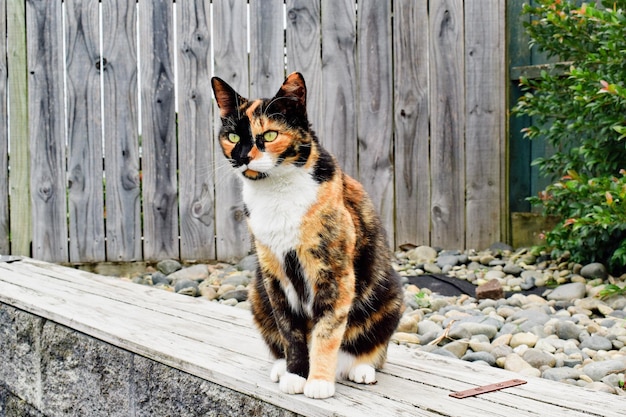A black-and-orange patterned tiger calico cat with distinct white patches on its chest, paws, and around its mouth sits in the center of the image. The cat is perched on a wooden-topped, stone wall with weathered, light grey stones streaked with dark grey, appearing dirty and mildewed. The wood panels of the wall, running horizontally across the image, are a pale ash-to-white color with a rusty metal strap on the right-hand side. Behind the cat, the back two-thirds of the image are filled with varied colored rocks, including beige, light grey, and pieces of old red bricks. Among the rocks is a black feather. To the right, a thin vertical strip of green bush with a few orange leaves is visible. On the left behind the cat, vertical wood paneling of a darker ash color forms a fence, with small gaps revealing daylight and some underlying bushes. The cat sits alert with its eyes open and ears raised, intently gazing towards the left, as if spotting something of interest.